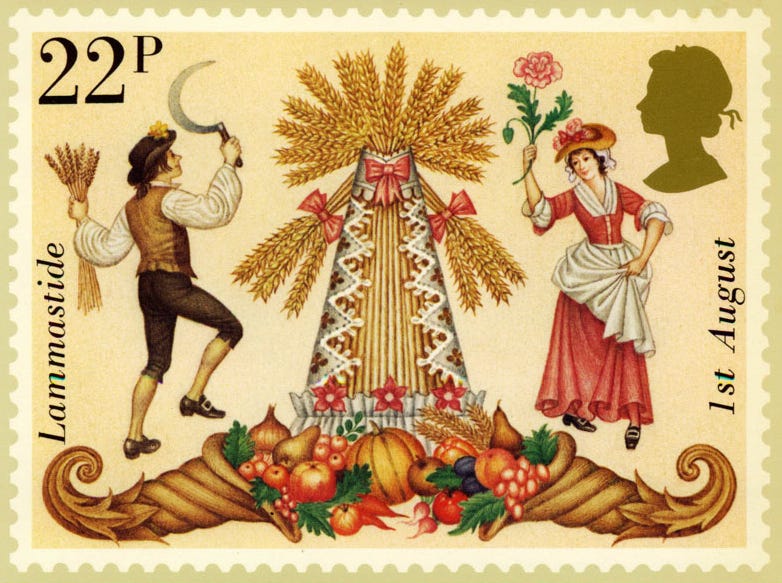This image features a vintage 22 pence stamp with a harvest season theme. The horizontally oriented stamp has a notched white border with a beige background. At the center of the stamp, a detailed illustration depicts a man and a woman. The man is holding a sickle and a bundle of wheat, while the woman, dressed in a red dress, is holding a rose stem and dancing. The scene includes a stack of hay adorned with pink ribbons, resembling a figure with arms, a headdress, and a white dress. Below, two cornucopias overflow with pumpkins and other vegetables. The stamp is labeled "22P" in the upper left corner, "1st August" on the right, and "Llamastide" on the left.